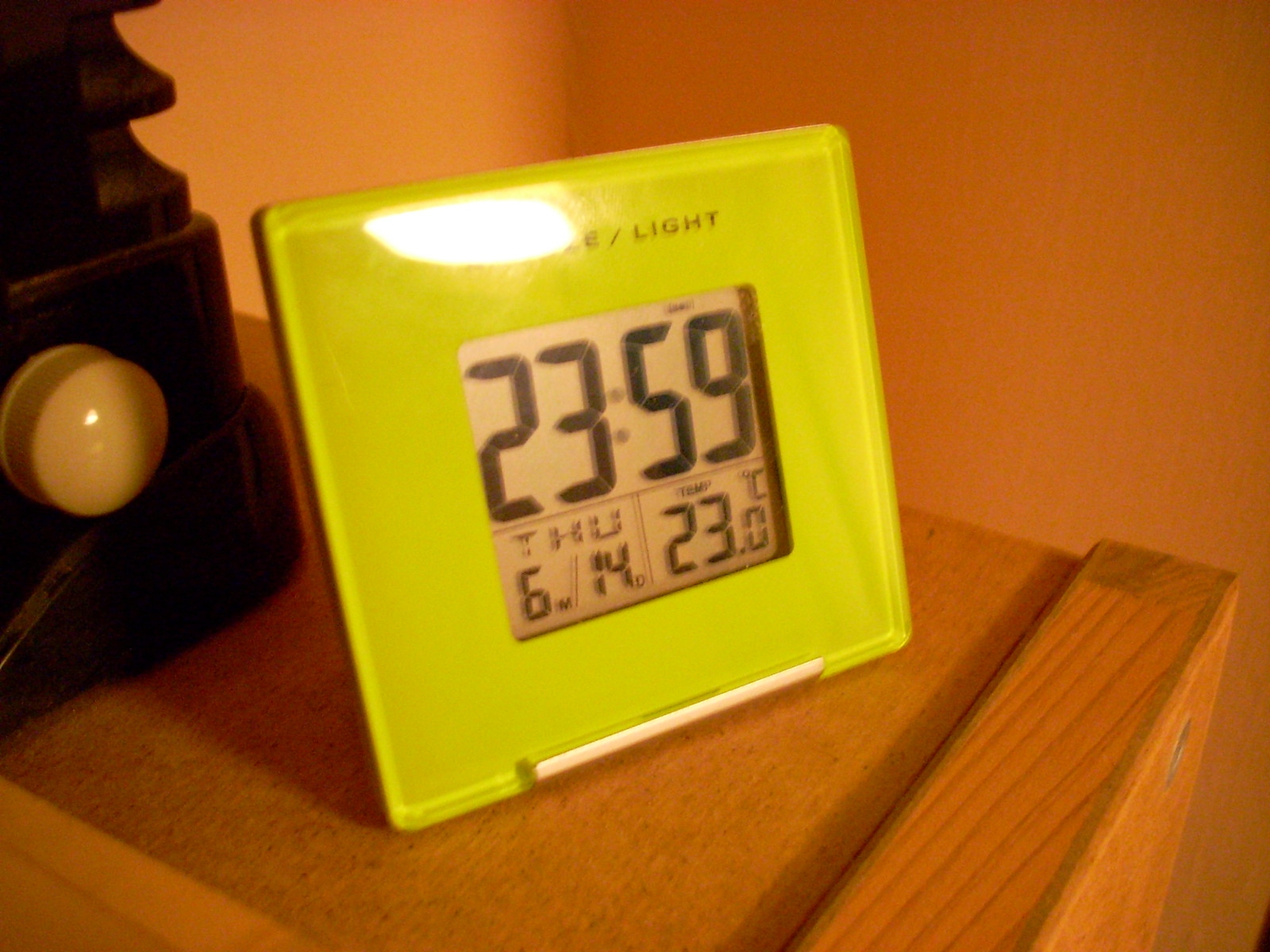A modern, rectangular digital alarm clock takes center stage in this photograph. The clock, a vibrant chartreuse, is positioned on a light wood end table. The screen of the clock displays the time as **23:59** in a black font against a light tan background. Above the time, there is an unreadable small word, partially obscured by a white oval caused by a light reflection. The clock's face also features the day "THU" for Thursday, the date "6M/14D," and the temperature, which reads "23.0°C." The upper part of the clock shows the word "light" in black lettering following an obscured section a slash mark. 

Behind and to the left of the clock rests a mysterious black unit with a white knob, creating a contrast against the light peach-colored wall in the background. This setup enhances the bright and clean aesthetic of the scene, highlighting the modern design of the alarm clock against the warm and subtle tones of the surrounding environment.